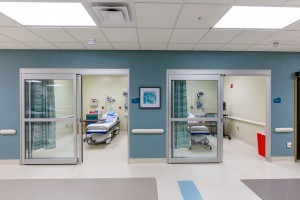This is a full-color photograph of a medical facility, likely a hospital emergency room or urgent care center. The image, taken indoors with artificial light, shows two adjacent observation rooms separated by a wall. Each room features an open full-length sliding glass door with silver trim and a blue privacy curtain that can be pulled across. 

The ceiling is composed of standard gray tiles with a central vent and two large fluorescent lights. The walls are painted blue, and there is a picture hanging on one of them, though its details are unclear. The floor is covered in light gray or whitish tiles interspersed with darker gray and bluish areas.

Inside each room, there is a hospital bed and various standard medical equipment, including devices for measuring blood pressure and red plastic bins for disposing of hazardous materials.